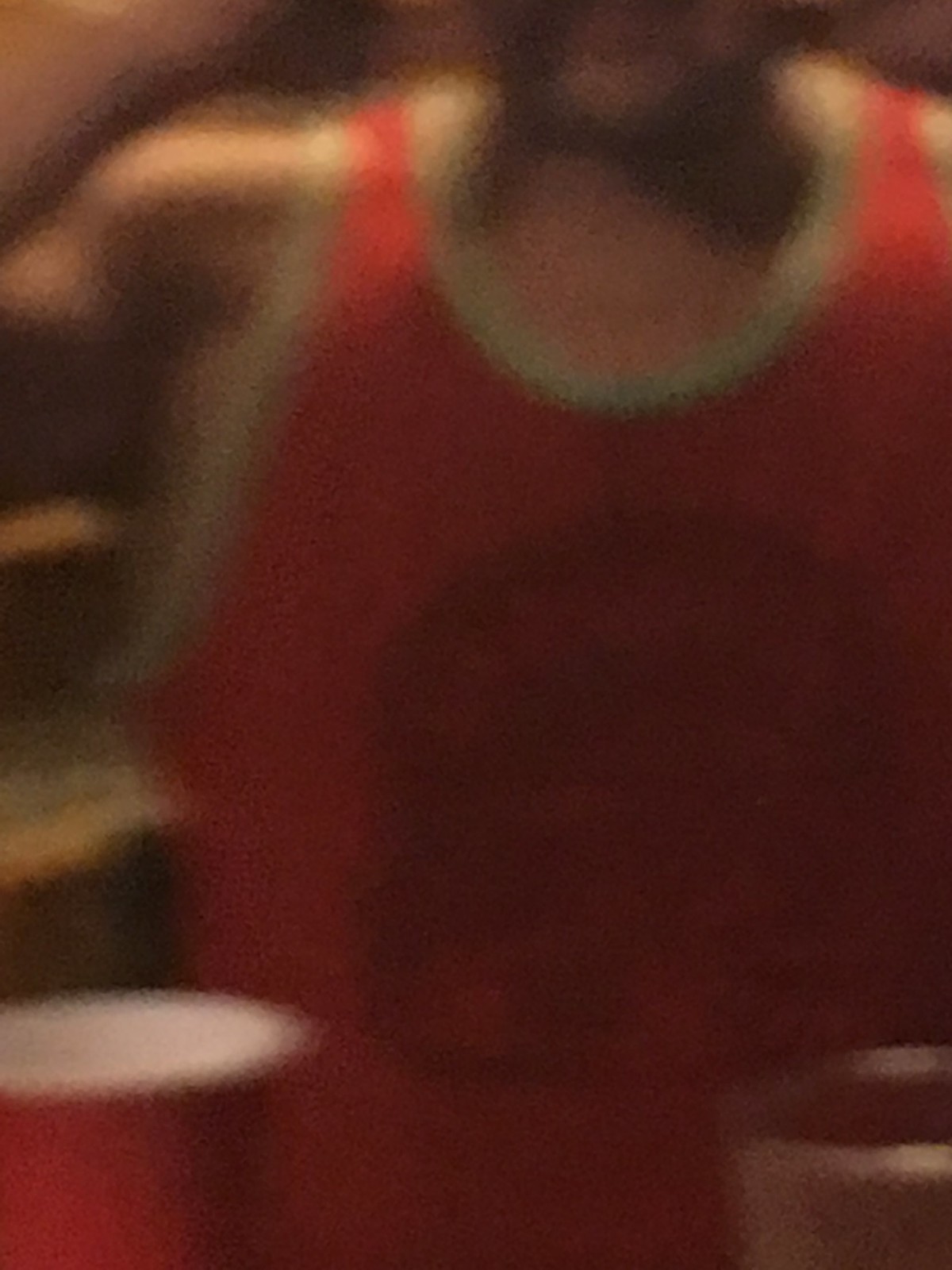An extremely out-of-focus photograph featuring a chaotic yet intriguing scene. In the bottom left corner, a red paper cup with a white interior stands prominently. To its right, there's a clear plastic cup. Dominating the majority of the image is what seems to be a man's red muscle t-shirt with white trim around the neck and armholes, his right shoulder and arm partially visible. His neck and a hint of his left shoulder can also be discerned. The man sports a black beard, with just a snippet of his chin captured. Adding to the mystique, there's an indistinct black design on the red t-shirt.